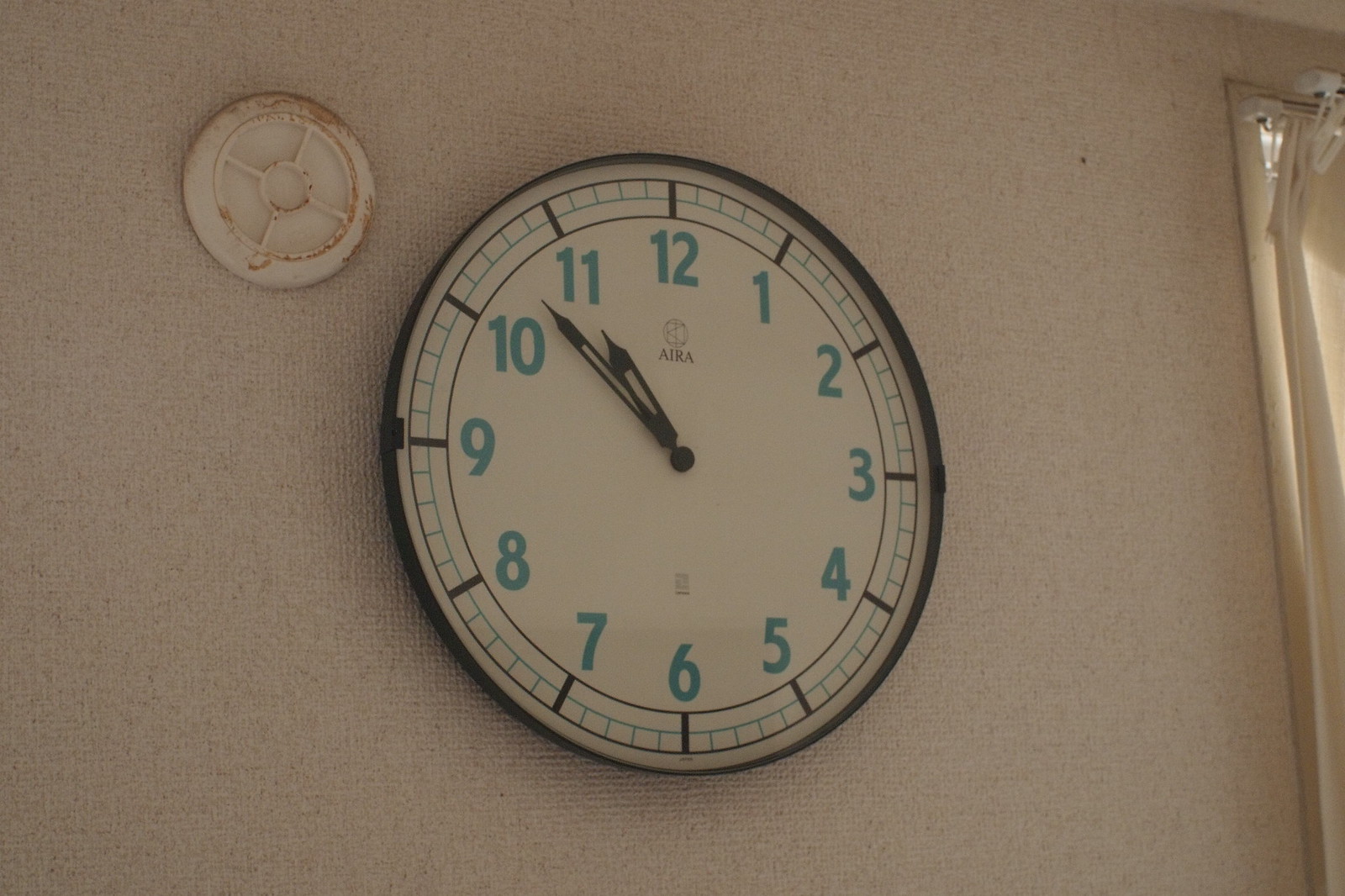In this photo, we see an analog clock mounted on a beige wall. The clock has a black outer rim and features teal numbers ranging from 1 to 12. The clock hands are designed like arrows with rectangular gaps, adding a touch of elegance. The time displayed is approximately 10:53. The photo quality suggests it was taken with an older camera or phone, as it's not very sharp.

To the right of the clock, part of a window is visible, covered by beige curtains that allow some light to filter through, indicating it's likely taken during the day. To the top left of the clock, there is a dirty, circular object on the wall that resembles a smoke detector, stained from what looks like years of exposure to smoke. The clock face also bears the text "A-I-R-A" along with a small symbol, possibly a watermark or logo.